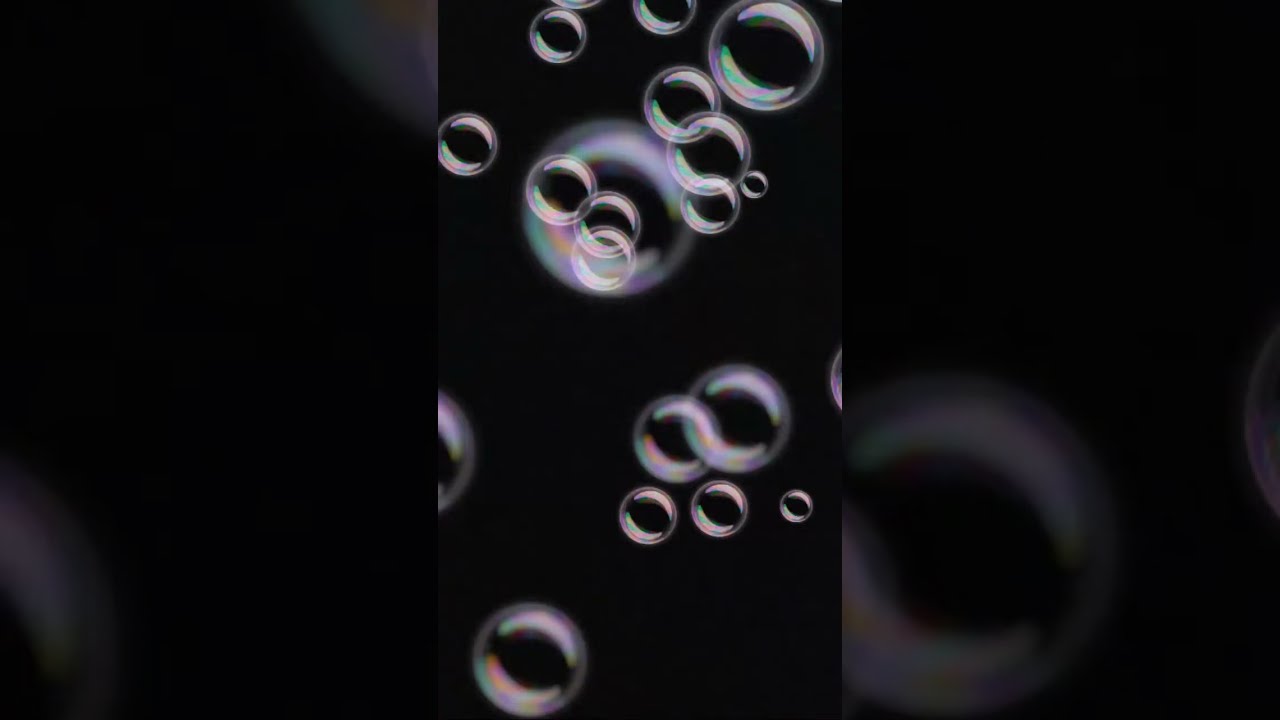This image features a dynamic and intriguing visual of soap bubbles set against a stark black background. The central portion of the composition, oriented portrait-style like a mobile phone display, showcases a collection of photorealistic bubbles. These bubbles vary in size and appear highly detailed with identical reflections, giving a copied-and-pasted effect. Surrounding this central image, on the left and right, are blurred and zoomed-in fragments of the same bubble photograph, reminiscent of an HDTV layout. The overall shape of the image is wider than it is tall, similar to a high-definition TV screen, creating a sense of depth. There are approximately fifteen bubbles in total, scattered throughout the image, from the top to the middle, and a few drifting towards the bottom. This arrangement of floating, misty bubbles in motion enhances the ethereal quality of the photograph, and the absence of any text and human figures adds to its simplicity and focus on the bubbles' delicate beauty.